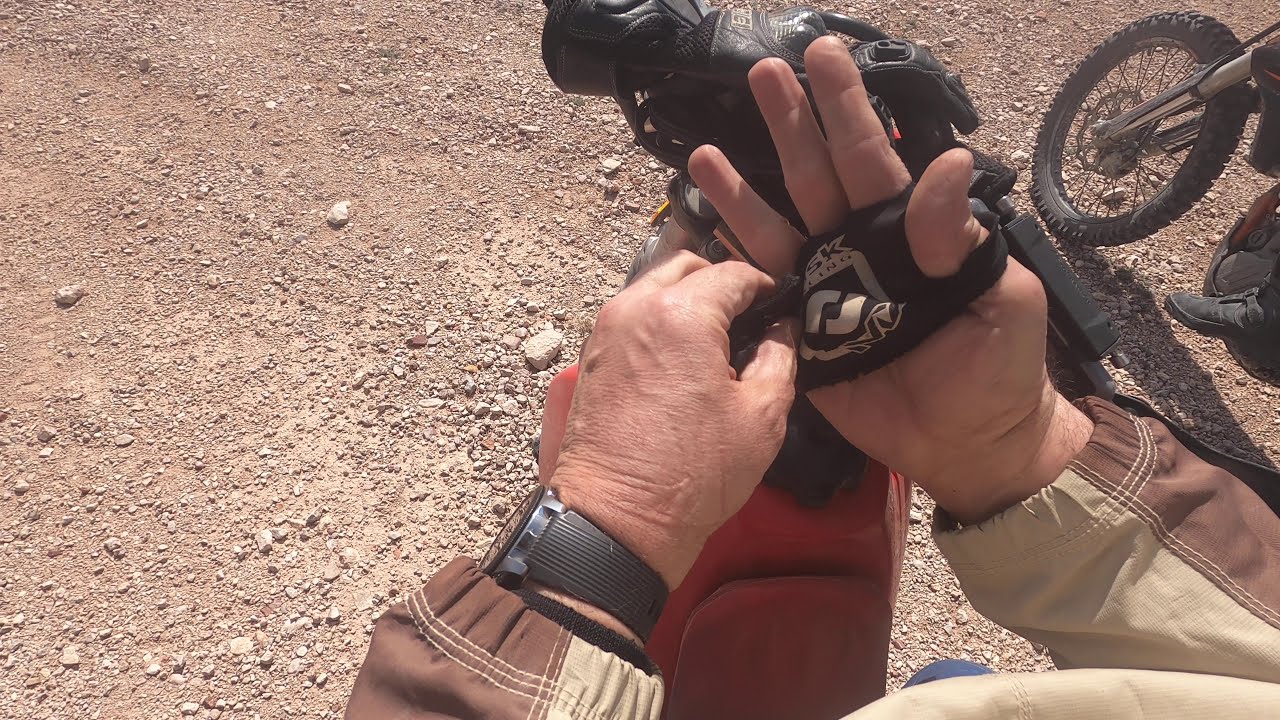The image depicts an outdoor scene with a dry, brown dirt surface covered in tiny stones. At the center of the image, a person, likely a man, is wearing a brown and beige jacket and is in the process of putting on a black fingerless glove with a white pattern. His left hand aids the right in pulling the glove over the fingers. A black watch is visible on his left wrist. To the right of the image, part of a red motorcycle or dirt bike is noticeable, including its wheel and a foot near it, suggesting that the person may be preparing for a ride. The overall setting appears to be a dirt bike trail on a clear day.